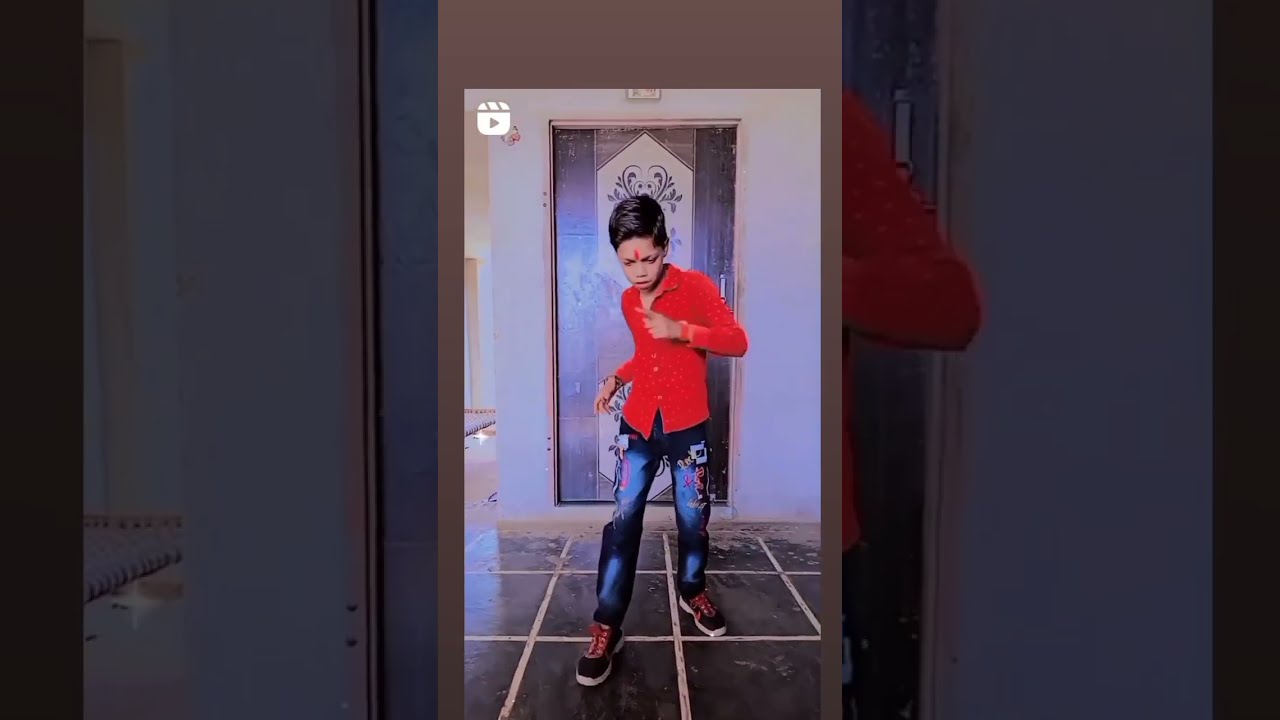The image features a young Indian boy, likely captured in a paused video, indicated by a play icon in the top left corner, suggesting it's a YouTube short or Instagram reel. The boy appears to be dancing, with his right foot forward and left foot back, exuding a sense of movement. He is dressed in a long, red button-down shirt and embroidered blue jeans featuring red and yellow floral patterns. His shoes are black with striking red laces. A distinct vertical red mark adorns his forehead, characteristic of cultural significance. The setting includes a large-tiled grayish floor beneath him, and behind him, a cream-colored wall with a white and brown door positioned at the center. The door has a fancy design, adding an elegant touch to the otherwise simple background. The whole image has a slight purplish-bluish tint, enhancing the visual appeal and creating a vibrant, lively atmosphere.